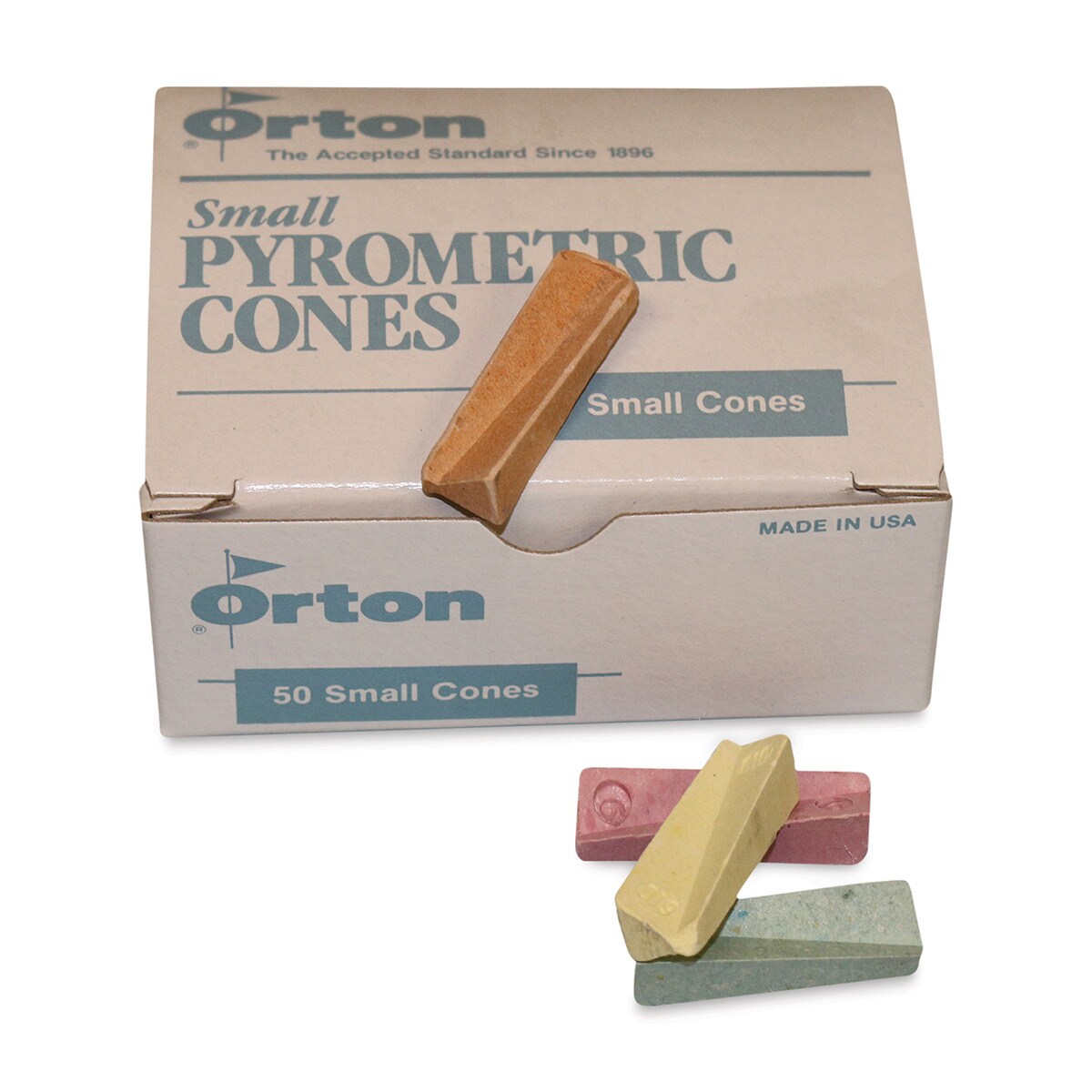The image features a light-colored, possibly waxed cardboard box from the Orton Company. The box prominently displays the Orton logo, which includes a triangular flag on a flagpole emerging from the first 'O'. Beneath this logo is the slogan "The accepted standard since 1896," written in a light blue or grey color. The box is labeled with "50 small pyrometric cones" on both the front and side panels, along with a statement in the top right corner that reads "Made in USA." The box is primarily tinted in shades of white and brown.

Accompanying the box are four small pyrometric cones. One brown cone rests atop the box while three more cones sit in front of it, arranged on a featureless white background. These front cones include varied hues: one is pink, another green, and the third is yellow, which intriguingly sits on top of the other two. This detailed and tidy arrangement clearly highlights the contents and branding of the product.